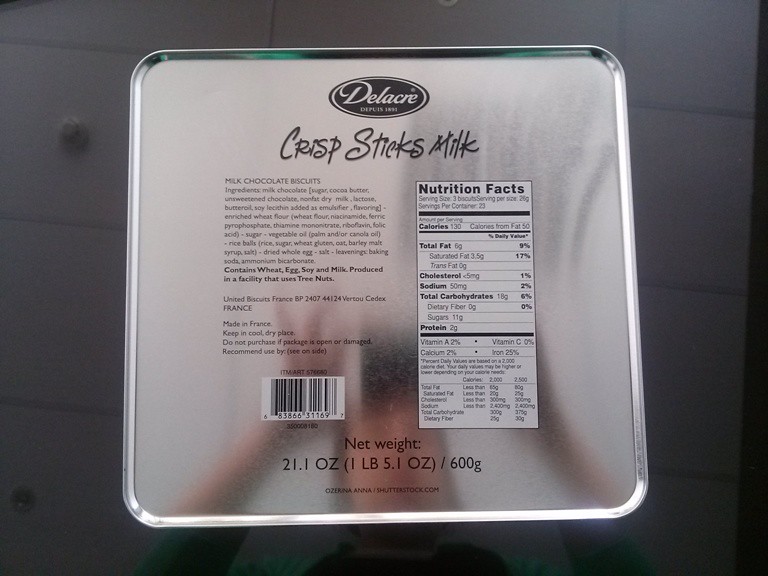The image depicts the bottom of a shiny, square metal tin package, reflecting a blurred image of the person taking the photo with their phone against a light gray, tile-like background. The tin features a chrome-colored outer ring that catches the light. At the top of the tin, within a black oval, the brand name "Delacre" is displayed in white cursive text. Below this, "Crisp Stix Milk" is written in black text. On the left-hand side, the ingredients are listed in very small black text, noting that the product contains wheat, eggs, soy, and milk, and is produced in a facility that uses tree nuts. Further down, there's an address indicating it is made in France, along with storage instructions and some additional information. On the right-hand side, within a white rectangular label, the nutritional facts are outlined in black text, detailing calories, total cholesterol, sodium, total carbohydrates, protein, and percentages for vitamins A, C, calcium, and iron. At the bottom, there is a barcode, a series of numbers, and the net weight listed as 21.1 ounces (1 pound, 5.1 ounces) or 600 grams.